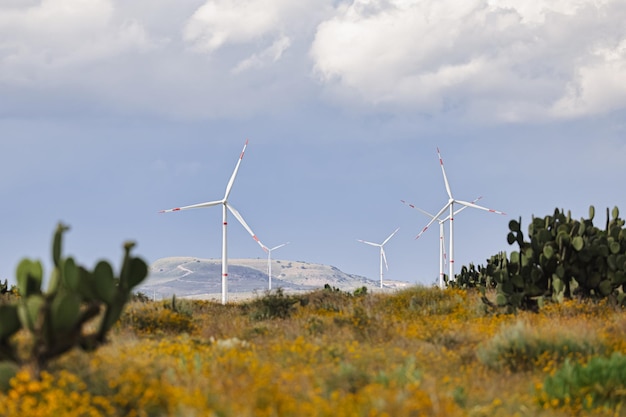The photograph showcases five tall windmills used for generating electricity, set against a desert landscape. The narrow, white barrel poles of the windmills extend straight up into the sky, each supporting three rotor blades that taper from thicker bases near the pole to narrower tips, accentuated with red stripes for visibility. The windmills form a pattern with three lined up consecutively on the right and two on the left. The arid terrain is dotted with green cacti and patches of yellow flowers, interspersed with clumps of orangish tumbleweed grass. In the background, there is a hill that seems partially covered with snow, adding a striking contrast to the desert flora. The sky above is a vivid blue adorned with puffy white clouds, suggesting it's daytime. This detailed scene likely captures a location in the mid to southwestern United States, emphasizing the juxtaposition of renewable energy technology within a rugged, natural environment.